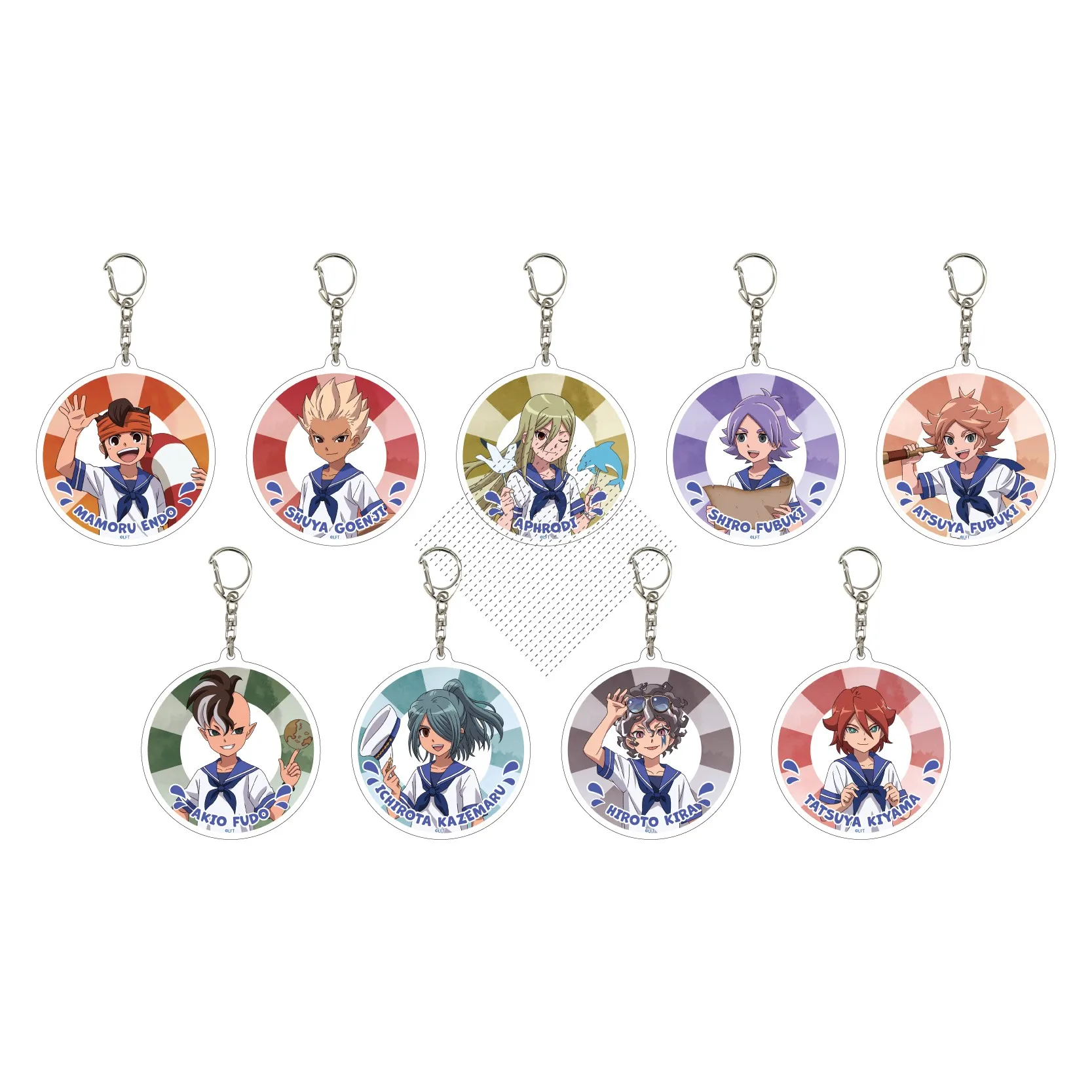The image showcases a collection of nine keychains, each featuring an anime character clad in a white sailor outfit with blue ornamentation. The characters vary by gender and have unique hair colors, including tan, green, blue, red, gray, and black. Each figure appears to be peering out from the middle of a life preserver, with their names displayed on the key tags in Japanese script. The keychains are attached to short silver chains with clasps, ideal for attaching to pockets or other chains. The backgrounds behind the characters vary, displaying an array of colors such as coral pink, mustard, olive green, violet, lavender, tan, and various shades of blue and red. The uniform design of white sailor tops paired with these vibrant backgrounds and hair colors makes each keychain distinct yet harmonious within the collection.